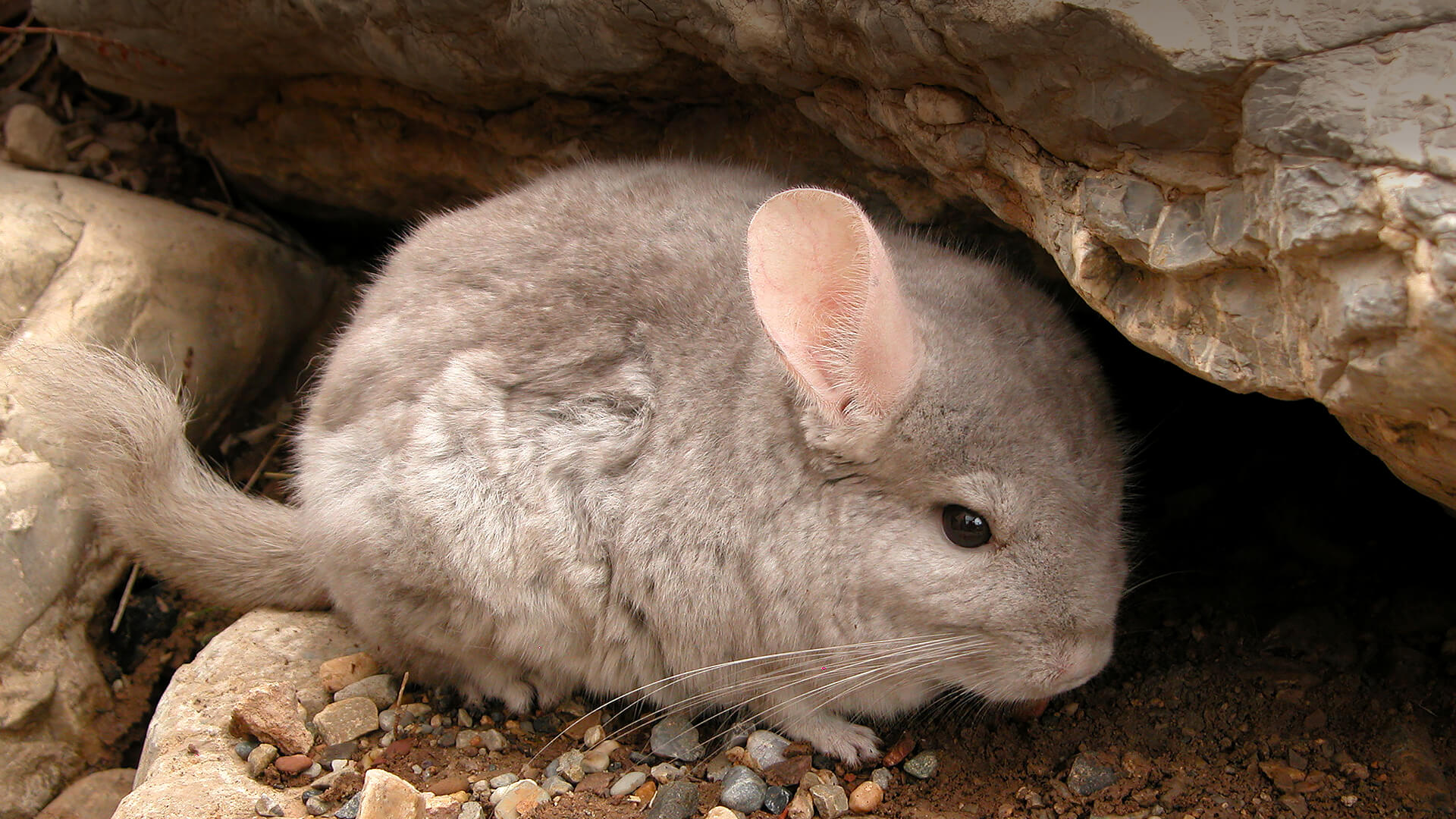This is a close-up photograph of a furry gray chinchilla nestled within a crevice of a rock wall. The rock formation around it is tan and light brown, with dark brown dirt and small pebbles scattered on the ground. The chinchilla's body is light gray, and it has distinctive pink ears, although only one is visible. Its black eyes, long white whiskers, and thick, bushy gray tail stand out prominently. The chinchilla is shown in full side profile, highlighting its round, plush body and tiny little paws. The background includes a predominant gray boulder with a sharp edge and a dark cavity, adding depth and context to its natural habitat. The image captures the subtle colors of gray, light pink, and varying shades of brown, bringing out the texture and details of both the animal and its surroundings.